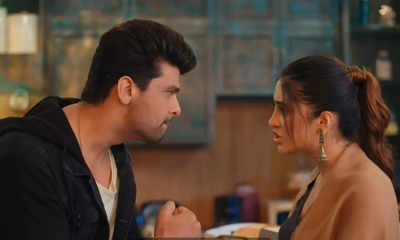This photograph, seemingly a still from a TV show or movie, captures an intense argument between a man and a woman set in what appears to be a kitchen. The man, positioned on the left, has short dark hair styled in a greaser pompadour and wears a dark black bathrobe over a white shirt, giving off a tough, perhaps mobster-like aura. He is visibly angry, clenching his fist and sporting an unshaven look. Opposite him, the woman, who bears a resemblance to Jennifer Lopez, is dressed up in a tan blazer, with her hair neatly pulled back and accessorized with earrings. She is speaking, her mouth open, trying to explain something with a serious yet intense expression. The background features wooden cabinetry and a shelf holding jars and other kitchen items, all set against a dimly lit ambiance that accentuates the tension of the scene.